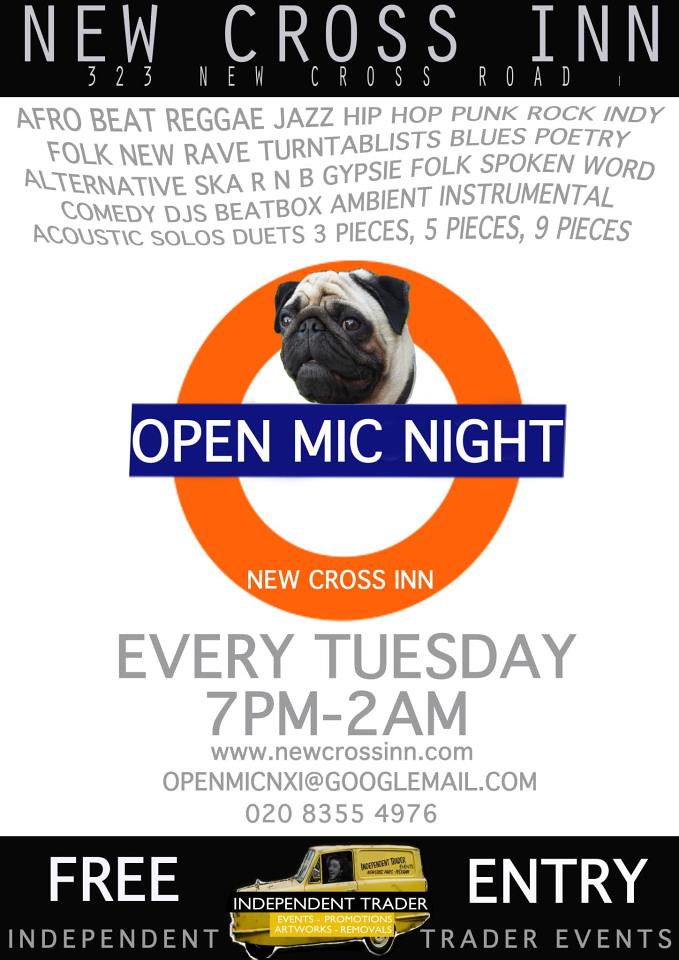This image is an online flyer for an Open Mic Night event at the New Cross Inn, located at 323 New Cross Road. At the top, a black banner prominently features "New Cross Inn" followed by the address. Below this, set against a white background, there's a wide array of genres listed in grey text with a slight psychedelic swirly effect: Afrobeat, Reggae, Jazz, Hip Hop, Punk, Rock, Indie, Folk, New Wave, Turntablist, Blues, Poetry, Alternative, Ska, R&B, Gypsy, Folk, Spoken Word, Comedy, DJs, Beatbox, Ambient, Instrumental, Acoustic, Solos, Duets, 3 Pieces, 5 Pieces, 9 Pieces. Below the genre list, a design element includes an orange circle containing the face of a beige pug, with black eyes and nose, overlaid by a blue banner reading "Open Mic Night" in white text. Details follow indicating the event occurs every Tuesday from 7 PM to 2 AM, with contact information including the website (www.newcrossinn.com), email (openmicnxi@googlemail.com), and phone number (020-8355-4976). At the bottom, another black banner states "Free Entry," accompanied by an image of a yellow taxi labeled "Independent Trader Events, Events, Promotion, Artwork, Removal."